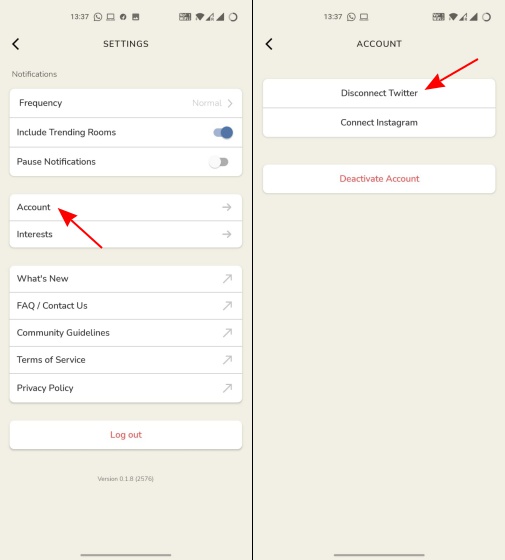The photograph features two screenshots from a mobile device, both with a beige background and captured at 13:37 military time. Indicators of Wi-Fi and carrier signals are visible at the top of each screen.

The left screenshot displays the "Settings" menu, recognizable by a black back arrow. Within the "Notifications" section, there is an option labeled "Frequency," which can be expanded. Notably, the "Include trending rooms" option is activated, indicated by a toggled-on blue switch. In contrast, "Pause notifications" is toggled off. There are subsections for "Account" and "Interests," each marked with red arrows indicating further details can be accessed. Additional menu items include "What's new," "FAQs and Contact us," "Community guidelines," "Terms of service," and "Privacy policy." At the bottom, a "Logout" button is present.

The right screenshot shifts focus to the "Account" settings. Here, options such as "Disconnect Twitter," pointed to by a red arrow, "Connect Instagram," and "Deactivate account" are listed. The "Deactivate account" option is particularly prominent, displayed in red text. The same Wi-Fi and carrier signals are present at the top of this screenshot as well.